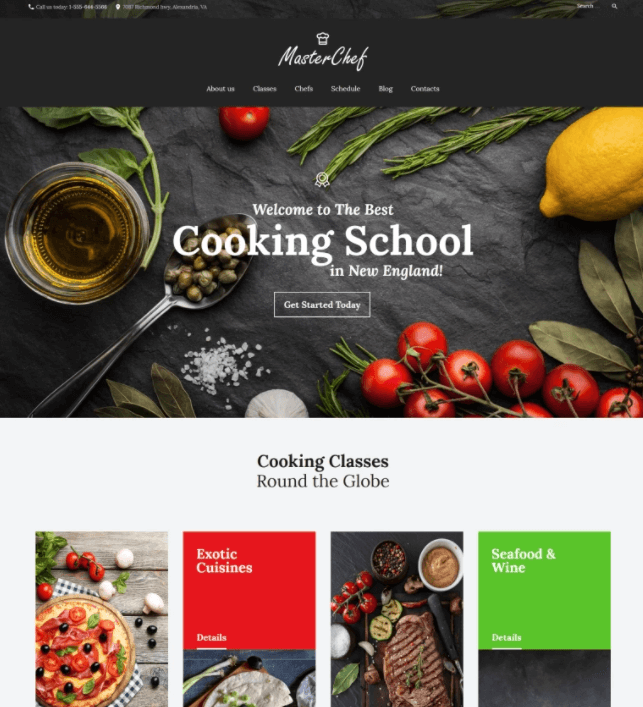The web page for the restaurant "MasterChef" features a sleek black header with the restaurant's name prominently displayed in the center, accompanied by a classic white chef's hat. The navigation bar beneath includes tabs labeled: About Us, Careers, Chefs, Classes, Schedule, Blog, and Contacts.

Below the header, a large dark gray rectangular section showcases a culinary arrangement. On the left, a small glass bowl contains balsamic vinegar with a distinctive yellow hue. Adjacent to the vinegar, a spoon holds a mix of light green beans interspersed with tan and dark green varieties. To the right, a cluster of tomatoes is accompanied by a sprinkle of salt and a sliced onion. Further to the right, a lemon adorned with dark green leaves adds a fresh citrus touch.

In the middle section of the page, a mid-gray box prominently displays the words "Cooking Classes" in bold black font, with the subtitle "Round the Globe" in a lighter, unboldened font below it. To the left of this section, a rustic wooden table is presented with a delectable homemade pizza topped with sliced tomatoes, dark green leaves, and black olives. Surrounding the pizza are white mushrooms that have yet to be integrated into the dish.

Next to this display, a striking large red rectangle captures attention with the title "Exotic Culinary" in bold white letters. Towards the bottom, the word "Details" introduces a section featuring a fajita wrapped with vibrant greens. Nearby, a perfectly seared steak with grill marks is paired with a white glass bowl and a black glass bowl filled with red and black seasonings. Alongside these items are additional tomatoes and grilled cucumber slices.

On the far-right side, a predominantly green box with white text highlights "Seafood and Wine." Beneath this, the word "Details" sits above a black rectangle, inviting guests to explore more about this enticing offer.